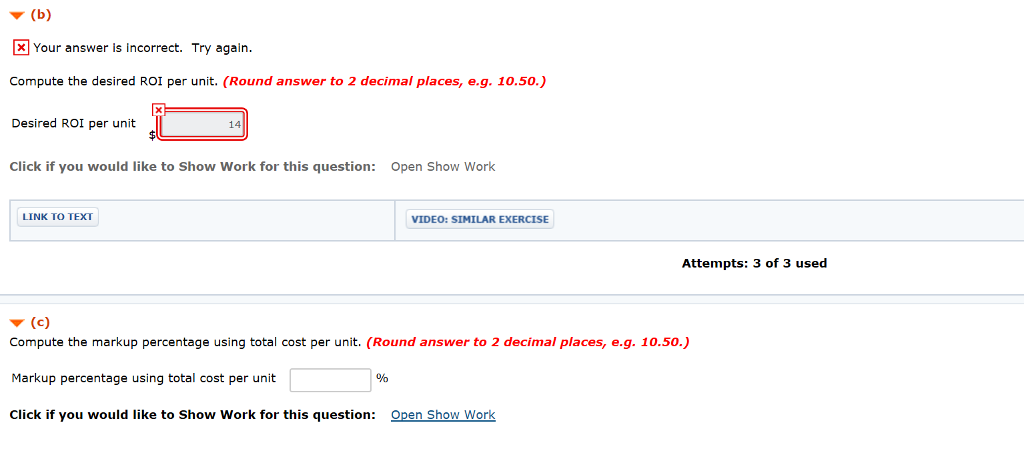The image is a horizontally rectangular screenshot with a primarily white background, depicting a section of an online test interface. 

At the very top, in red text, there's a lowercase "b" in parentheses with a downward arrow to its left, indicating the current question part. Directly below this, a red outlined box with a red X at its center alerts the user: "Your answer is incorrect. Try again."

Following this notification, the user is prompted to "compute the desired ROI per unit." A supplementary instruction in red, within parentheses, specifies: "Round answer to two decimal places, e.g., 10.50."

Directly beneath, there's a label "Desired ROI per unit" aligned beside a red outlined text field that contains the incorrect input "14." Below this field, a clickable option reads: "Click if you would like to show work for this equation." Adjacent to these instructions are two buttons labeled "link to text and video" and "similar exercise." 

On the right side, there's an indication of "Attempts: 3 of 3 used," signaling that the user has exhausted their attempts. Following this, the next part of the test question is marked with a lowercase "c" in parentheses, again paired with a downward arrow on the left.

The subsequent task instructs the user to "compute the markup percentage using total cost per unit," specifying again to "Round answer to two decimal places." This is accompanied by an empty input field designated for the markup percentage, with a percentage sign (%) placed to the right of the field. Lastly, a similar prompt appears: "Click if you would like to show work for this question."